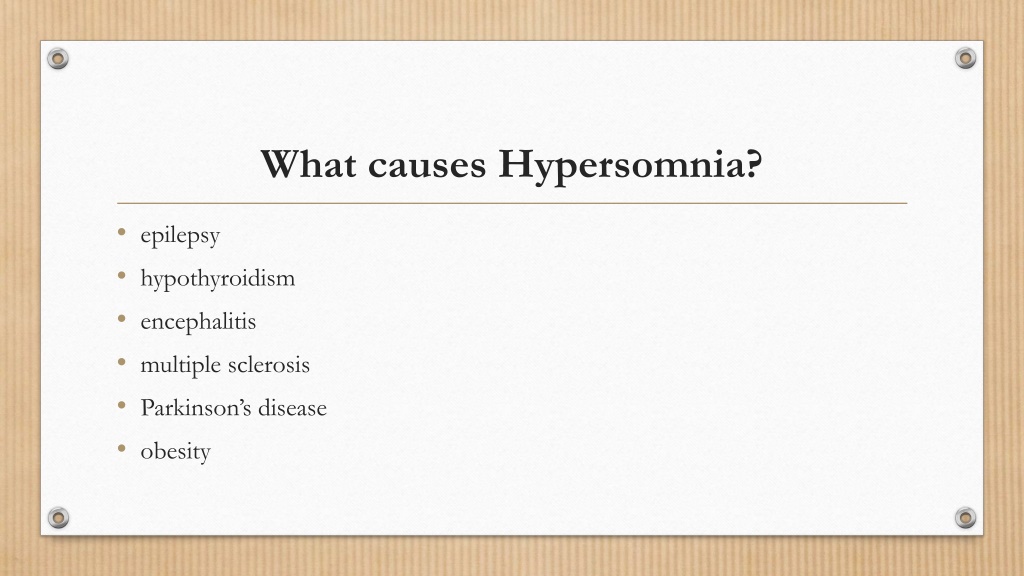In this detailed image, we observe a rectangular card with a brown background adorned with vertical lines running throughout. Superimposed on this background is a white rectangle serving as a pop-up text box. Positioned at each corner of the white rectangle are four icons symbolizing males. At the top of the white rectangle, in bold black text, is the question "What causes Hypersomnia?" centered and prominently displayed. Beneath this question, a thin horizontal line stretches from left to right, dividing the question from the list of causes. The listed causes of hypersomnia, presented in black text, include:

1. Epilepsy
2. Hypothyroidism
3. Multiple Sclerosis
4. Encephalitis
5. Parkinson's Disease
6. Obesity

The layout and presentation suggest that this image is part of an app designed for testing knowledge about medical conditions, potentially useful for studying or general knowledge enhancement.